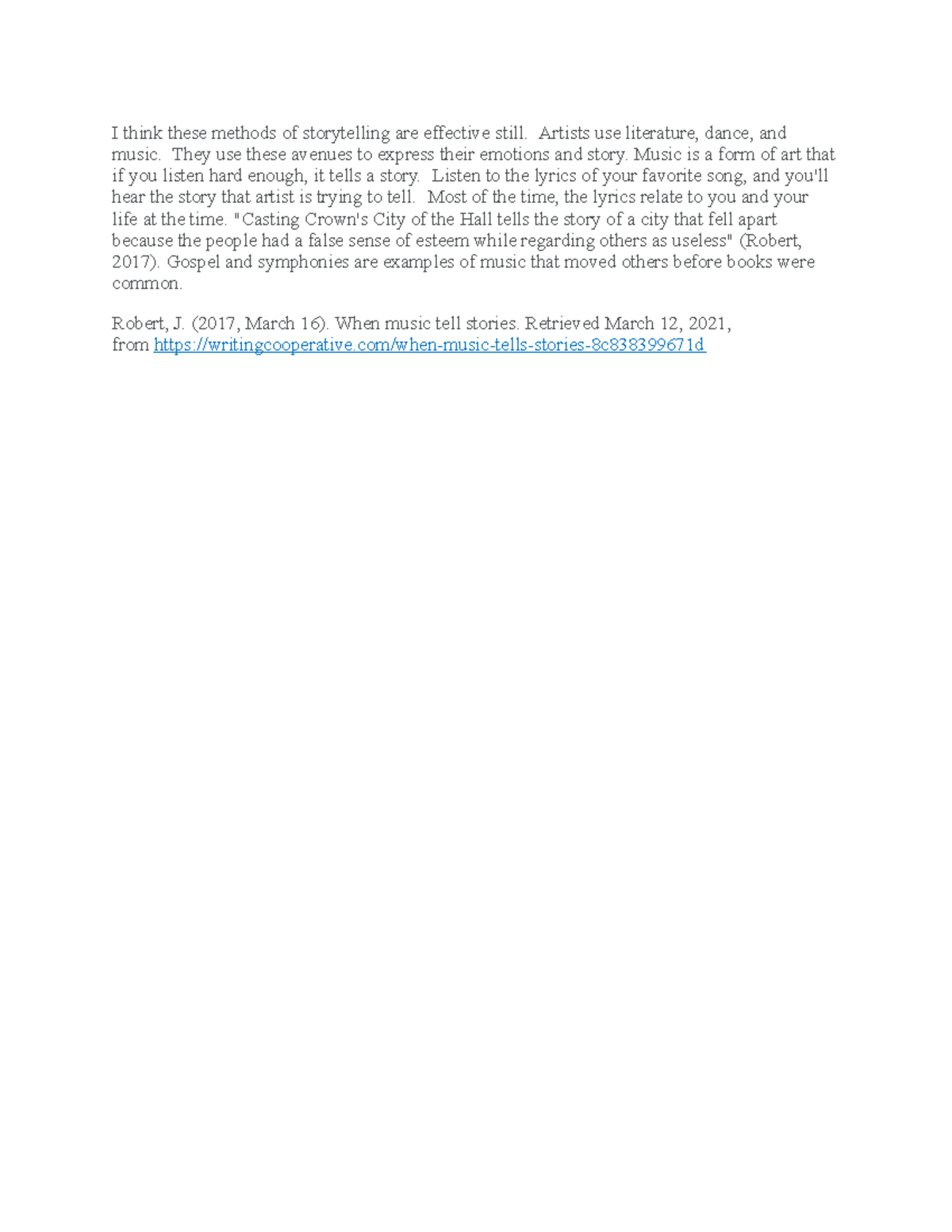This image captures a screenshot of text that originates from a Word document or a similar word processing page. The text is set against a plain white background and is presented in black, default Times New Roman font. The content appears to be an excerpt from an essay discussing the effectiveness of various storytelling methods. The passage states:

"I think these methods of storytelling are effective still. Artists use literature, dance, and music. They use these avenues to express their emotions and story. Music is a form of art that if you listen hard enough, it tells a story. Listen to the lyrics of your favorite song and you'll hear the story that artist is trying to tell. Most of the time the lyrics relate to you and your life at the time. Casting Crowns' 'City on the Hill' tells the story of a city that fell apart because the people had a false sense of esteem while regarding others as useless (Robert, 2017). Gospel and symphonies are examples of music that moved others before books were common."

At the end of the text, a reference is included: "Robert J., 2017, March 16. 'The Music Tells Stories', retrieved March 12, 2021, from writingcooperative.com."

Based on the nature of the content, it seems to be part of an essay, possibly an introductory section, providing a sample of the full narrative exploring the connections between music and storytelling.